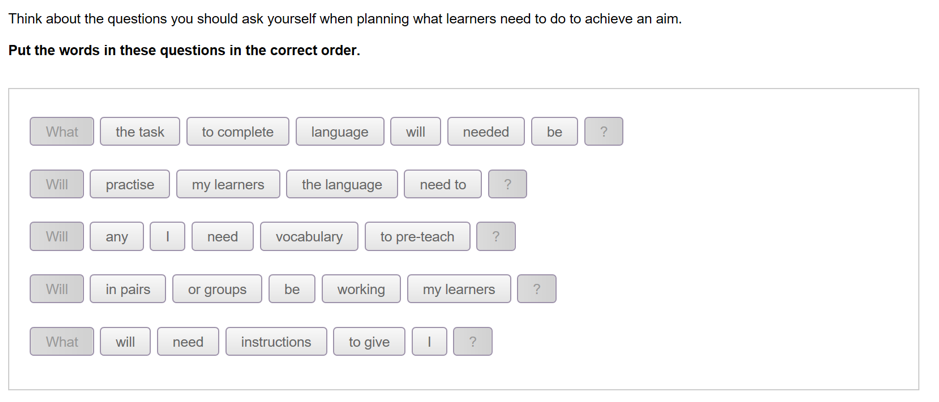In this image, a page is shown with a distinctive educational prompt, rendered against a stark white background. The center of the image features a light gray rectangular box that encases a series of words arranged in a button-like format. At the top of the page, a directive is prominently displayed in bold letters: "Think about the questions you should ask yourself when planning what learners need to do to achieve an aim. Put the words in these questions in correct order." 

Directly below this instructional text, there is a horizontal list of words distributed across five rows, resembling buttons. Each row comprises approximately seven to eight words, with slight variations in the number of words per row. The initial word in each row is highlighted in a slightly darker green shade for emphasis. The highlighted words are: "will," "will," "will," "what," and "what." Following these keywords, the remaining words stretch across the row, leading to a concluding question mark at the end of each row, signifying that these phrases are meant to be reordered into coherent questions.